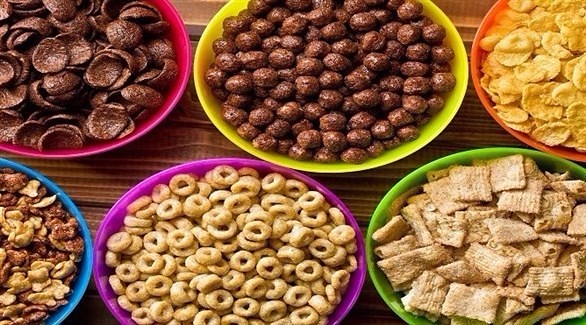This photograph is an overhead view of a dark brown wooden tabletop featuring six colorful bowls, each containing a different type of cereal. Starting from the top row, the top left corner has a red bowl filled with deep brown, curled-up disc-shaped cereal pieces. Next to it, a yellow bowl contains round cocoa puffs, characterized by their dark brown color. The top right features an orange bowl with light brown cornflakes.

In the bottom row, the leftmost bowl is blue and holds a mixed assortment of nuts and grains, resembling granola, with light and dark brown irregular pieces scattered with nuts. The center bottom bowl is purple, filled with beige ring-shaped Cheerios. Finally, the bottom right green bowl contains square pieces of Chex cereal, combining light and dark brown hues, likely indicating Cinnamon Toast Crunch-like squares with a smattering of darker tones.